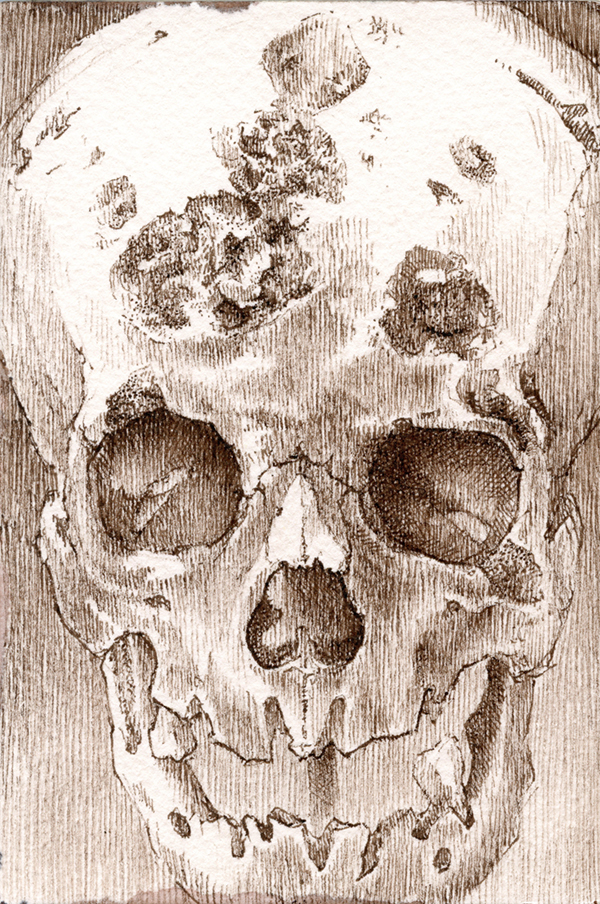This detailed artistic sketch features a large skull, prominently displayed with a variety of rich textures and tones. The skull, depicted in dark grey, brownish grey, and white, has a decrepit and hollow appearance, suited to a horror style. Its deep, empty eye sockets are shaded with cross-hatching to emphasize their dark, recessed nature. The nose is partially missing, presenting a large, whitish hole beneath it, while the toothless jaw forms a haunting, empty grin. The top of the skull is slightly cut off, revealing the sides curling around and showcasing a few dents and craters, especially three significant ones towards the middle and an additional one on the right side. The background features vertical lines, giving a textured, finely close-together look, reminiscent of fine-grain wood, alternating between dark and light areas. The entire image merges into a cohesive medical sketch, albeit with a graphic touch, heightening the eerie aesthetic with its meticulously shaded and textured details.